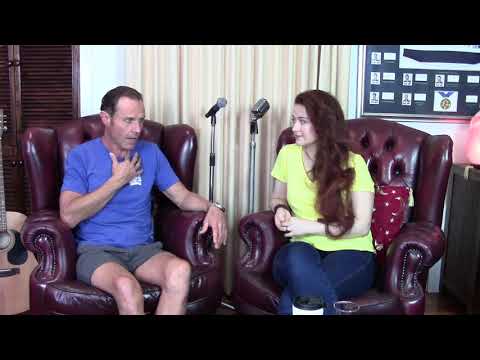In this detailed photograph, a man and a woman are sitting in red, leather recliner chairs, engaged in a conversation. The man, on the left, wears a blue shirt and gray shorts, with short brown hair. He is holding his right hand to his chest as if in mid-speech, while his left arm rests on the chair's armrest. The woman to his right has long, reddish-brown hair that flows down to her stomach and is wearing a yellow short-sleeve t-shirt and blue jeans, with her legs crossed. She sits on a pillow and appears to be listening intently to the man, her pale arms resting together in front of her. In between them, there are two silver microphones on stands. The background includes several elements: to the left, there is a closet with wooden double doors featuring a grid design, and nearby, an acoustic guitar is leaning against the wall. On the upper right side of the image, there's a framed portrait displaying people and several military or award medals. Additionally, a black shelving unit or bookcase is visible. This setup, complete with an off-white curtain in the background, suggests the space might be a rec room or studio. Black bars at the top and bottom of the image give it a letterboxed appearance.